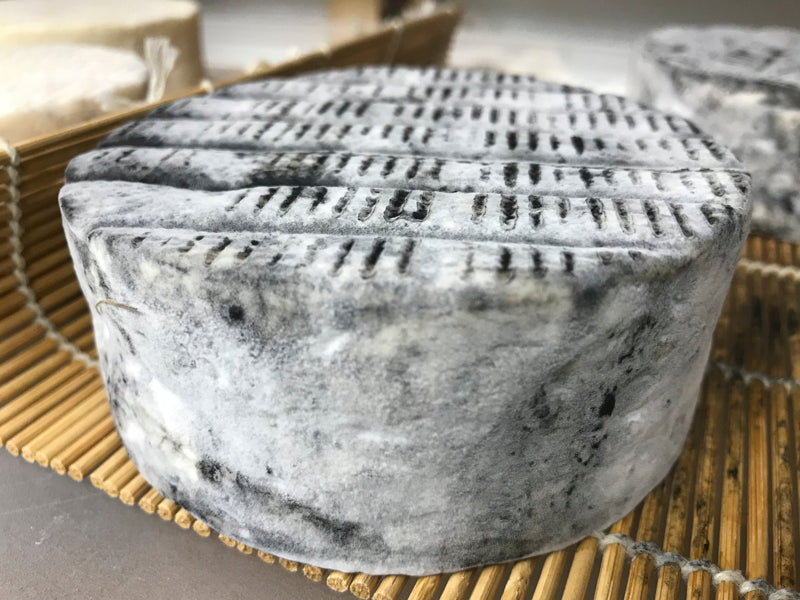The image features a meticulously detailed scene of a rustic kitchen setting. At the center of the composition is a thick, circular block of cheese, entirely enveloped in a gray, fuzzy mold with varying shades of lighter and darker gray. This moldy cheese rests upon a small wooden mat, constructed from numerous wooden sticks bound together, exuding an artisanal, hand-crafted aesthetic. Surrounding the focal cheese, additional cheese rounds can be seen; two in the upper left corner exhibit a healthy yellow hue, whereas another similarly moldy gray cheese is positioned in the top right corner. In the background, white pellets are scattered, adding to the textural complexity of the scene. Overall, the image captures a palette of gray, black, light brown, and white, contributing to an earthy, organic ambiance. The bamboo elements tied with rope, along with the various shades of mold and natural materials, collectively evoke a rustic, culinary-oriented setting.